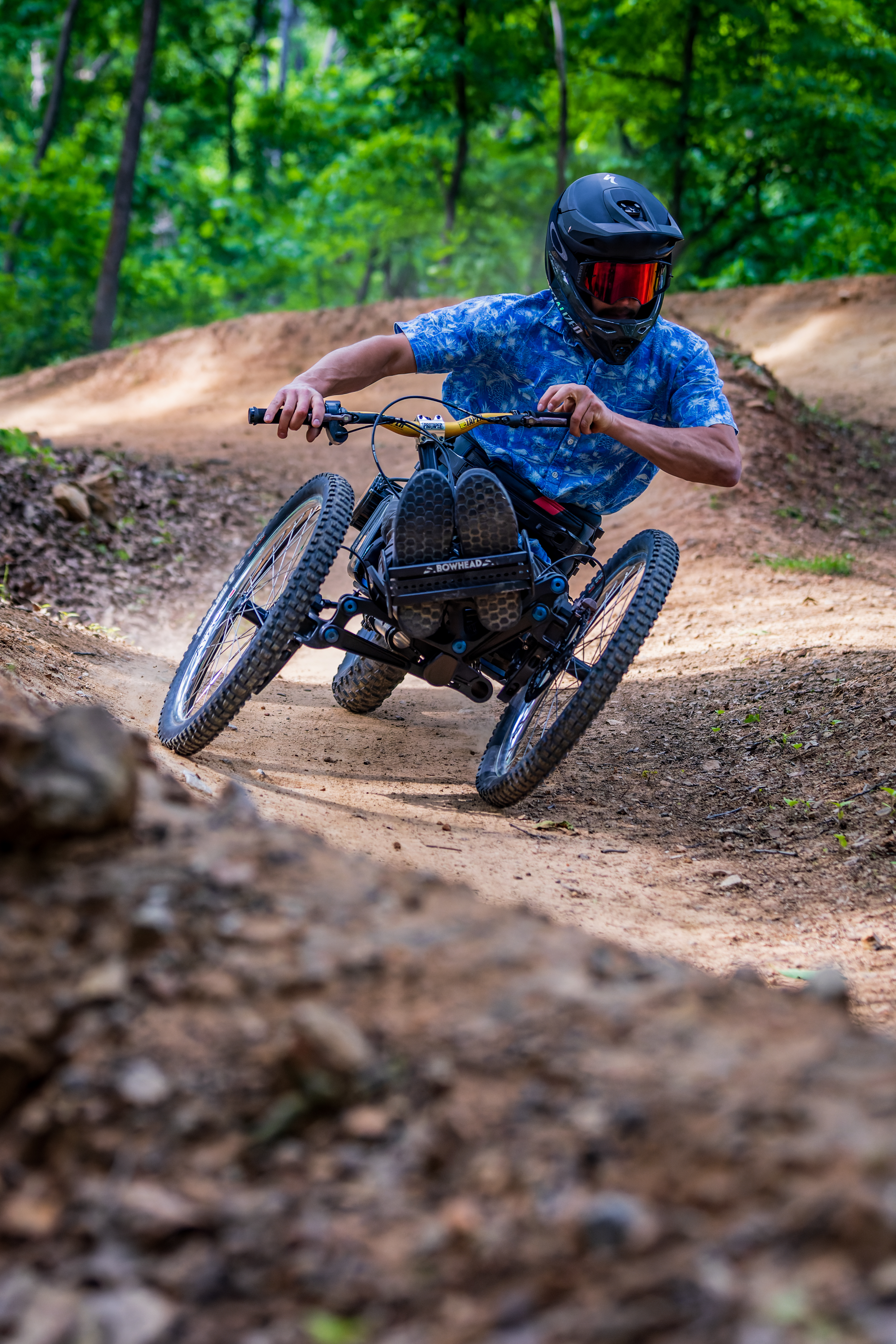In this photograph, a young man is racing down a dirt trail in a densely forested area, filled with vibrant green trees. He is riding a specialized three-wheel tricycle designed for disabled athletes, maneuvering exclusively with his hands on yellow and black handlebars. His legs are secured, elevated parallel to the ground. He is dressed in a short-sleeved blue shirt with white accents, dark-colored pants, and wears a black helmet with a reflective red visor, along with red protective glasses. Dirt is being kicked up behind him as he navigates a turn on the rugged track, indicating the intensity and speed of the competition.